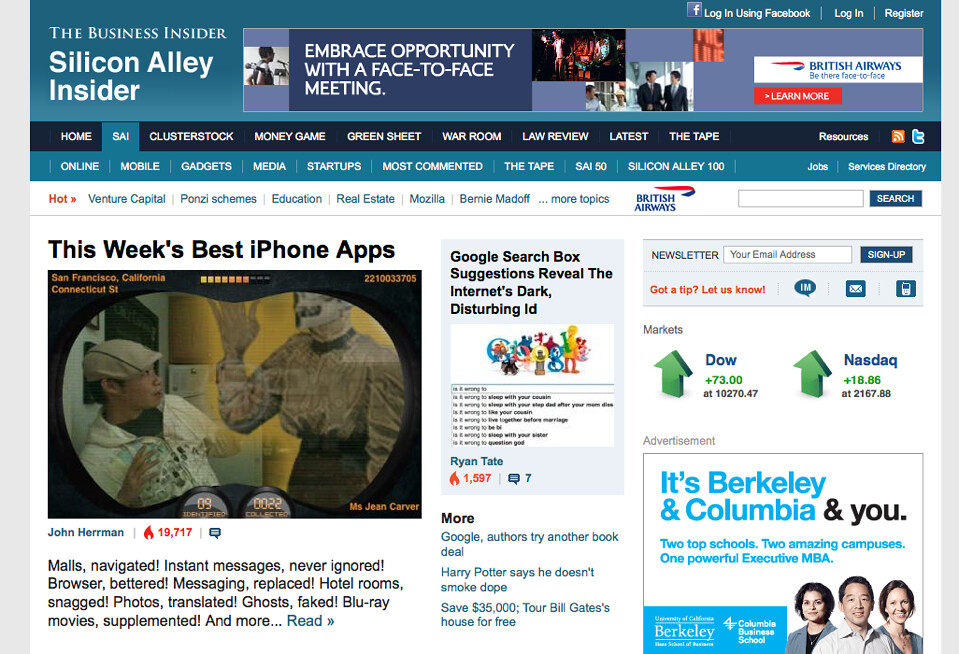This is a screenshot of a website with a primary focus on the "Business Insider" section. At the top, you can see a large grayish-blue rectangle. In the upper left corner of this rectangle, the text "Silicone Alley Insider" is displayed in white font. 

To the right of this title, there is a banner advertisement. The ad features the text "Embrace opportunity with a face-to-face meeting" in white font. The banner includes a series of small, random photos: one shows someone singing into a microphone, another features a person on a stage, and the last one depicts two men in suits sitting and talking to each other.

Next to these images, a white rectangle with the text "British Airways: Be there face-to-face" is present. Below this text, a red button with the words "Learn More" in white font invites users to explore further. Above this advertisement, the page provides options for users to "Login using Facebook," "Login," or "Register," all in white font. 

Beneath the advertisement section, a dark blue navigation bar contains several options in white font: "Home," "SAI," "Cluster," "Cluster Stock," "Money Game," "Green Sheet," "War Room," "Law Review," "Latest," "The Tape," "Resources,” and a Twitter logo. The user appears to have clicked on the "SAI" section.